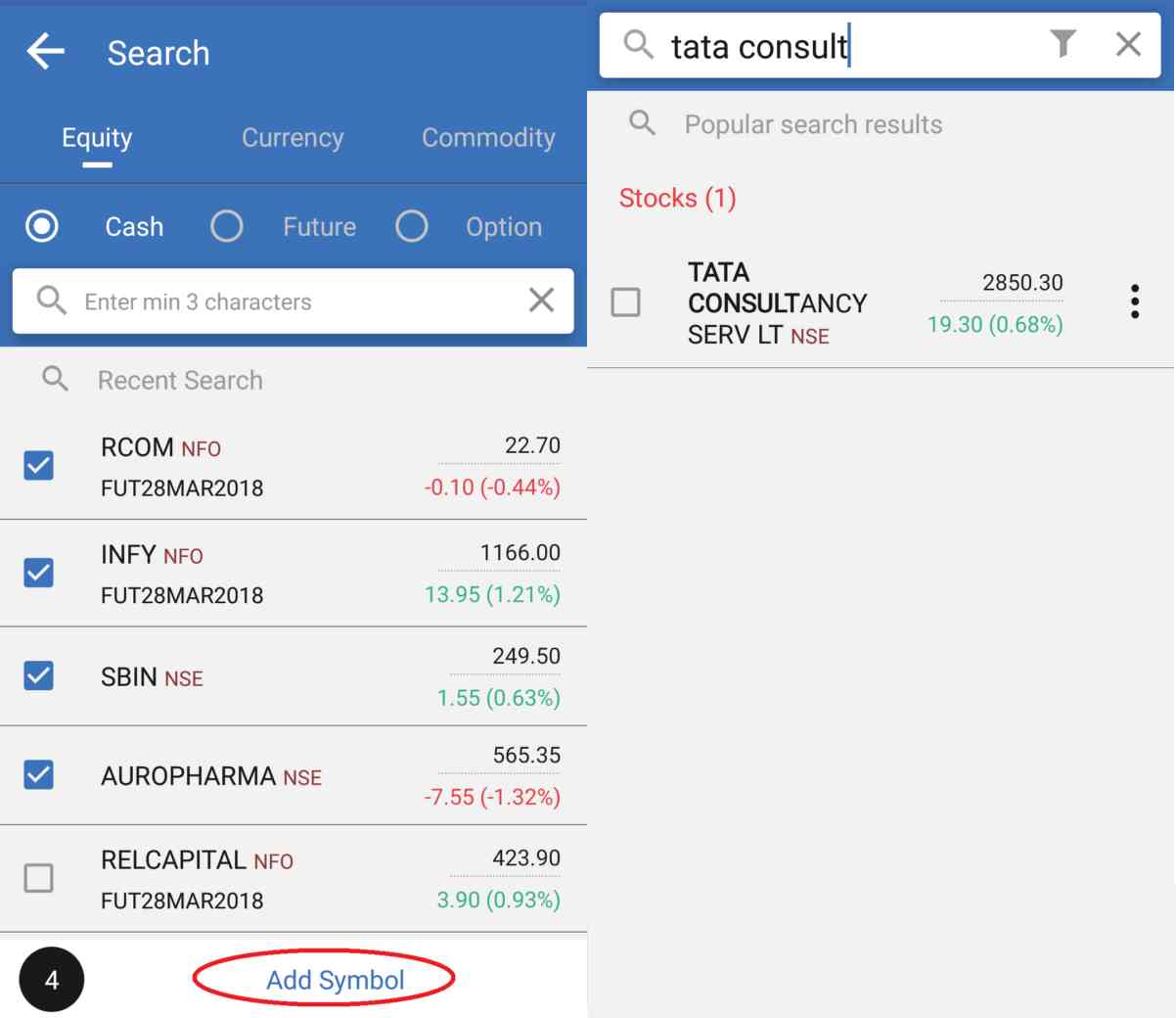This image showcases two screenshots of mobile applications with distinct interface designs.

On the left screenshot, the app features a blue header that includes a white arrow pointing left in the top-left corner, indicating a back navigation option. To the right of the arrow, white text reads "Search." Below this header, three white text options—"Equity," "Currency," and "Commodity"—are displayed horizontally, with "Equity" being underlined and appearing slightly brighter than the others, indicating it is the selected option. A thin dark gray line separates this section from another blue header below, which contains three more options each accompanied by a radio button on their left. The options are "Cash," which has a white circle with a blue outline and a thin white outline indicating selection, "Future," and "Option"—both represented by gray donut shapes that are not selected. Below these options, there is a white text box with a light gray magnifying glass icon on its left side and a light gray 'X' on the right, serving as a search bar. The body of the page has a light gray background. In the top-left corner of this section, there is a magnifying glass icon next to light gray text that reads "Recent Search." Below this heading, five rows of information are listed, each with a checkbox on the left. The first four checkboxes are filled blue squares with white checkmarks, while the fifth is just a medium gray outlined box. Each row of information features black text followed by smaller red text to its right: "RCOM" with "NFO" in red, "INFY" with "NFO" in red, and subsequent lines following similar formatting.

The right screenshot also features a light gray background and a blue header. At the top of this header, a prominent white search bar is centered, facilitating user input for searches. The design suggests continuity in the app's visual language through the use of consistent color schemes and text formatting.